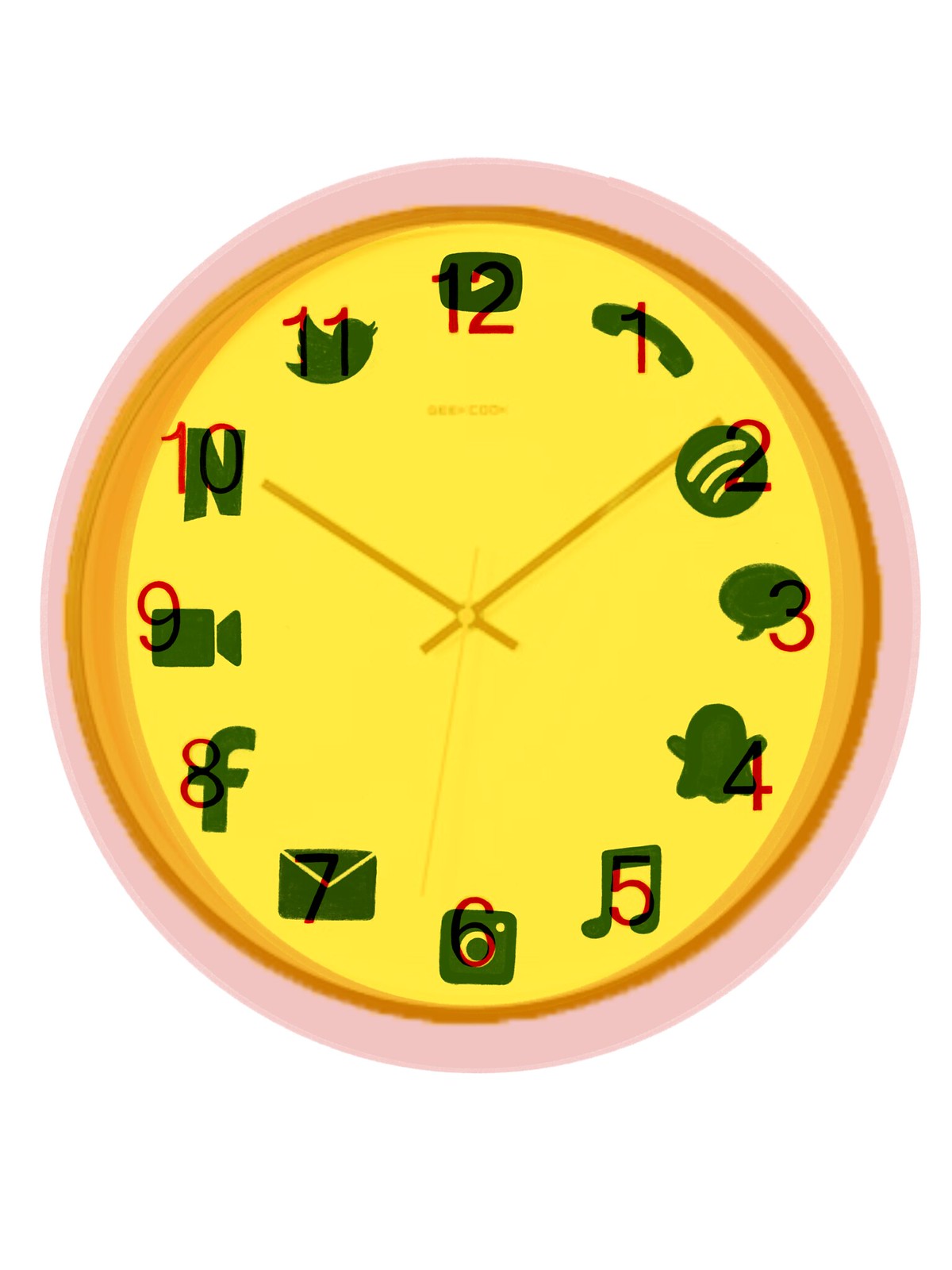This digitalized image features a highly unique clock with a striking color scheme and intricate details. The outermost rim of the clock is a soft light pink, followed by a darker yellowish-orange ring closer to the center, which transitions into a lighter shade. The clock's central face is a vivid, bright yellow.

The clock's hands are distinctively colored: both the hour and minute hands are a darker yellow, while the second hand is a lighter shade of yellow. The numerals marking the hours are bold red, running from 12 all the way around the clock face.

Above each numeral, there is a faint, overlaying symbol representing various popular mobile applications and platforms. Starting from the top and moving clockwise, the symbols include:
- 12: Phone icon
- 1: Spotify icon
- 2: Text message icon
- 3: YouTube icon
- 4: Snapchat icon
- 5: Music note icon
- 6: Instagram icon
- 7: Gmail icon
- 8: Facebook icon
- 9: FaceTime icon
- 10: Netflix icon
- 11: Twitter icon

Each symbol is subtly faded yet recognizable, providing a modern and tech-savvy twist to the traditional clock design.